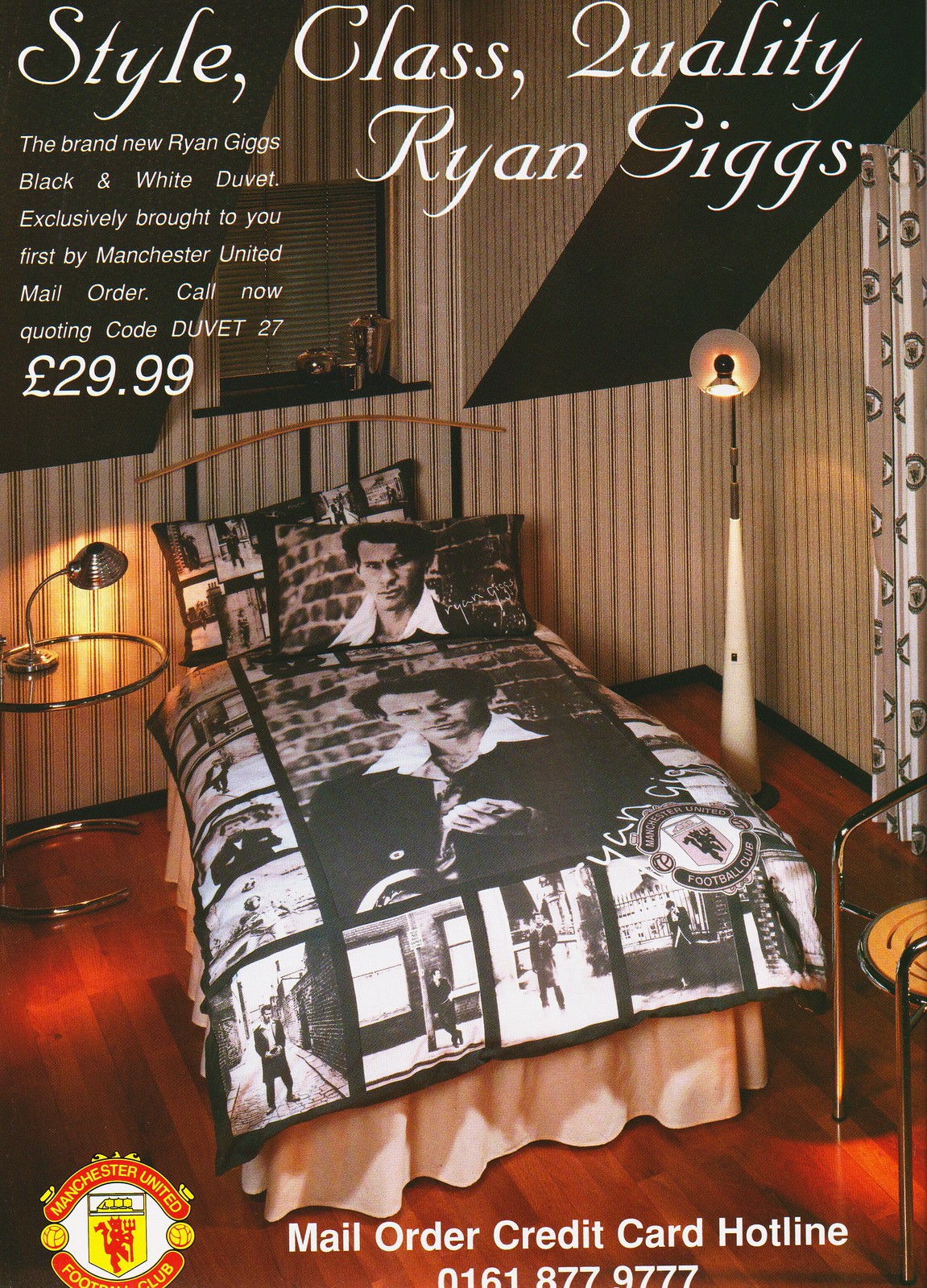The advertisement is a vertically-oriented image promoting the brand-new Ryan Giggs black and white duvet, exclusively available through Manchester United Mail Order for £29.99. The top of the image features the text "Style, Class, Quality, Ryan Giggs" in white script. Dominating the center is a photograph of a single twin bed dressed with the duvet, which showcases various black and white images of Ryan Giggs. Flanking the bed are two lamps, one on each side, and the wall behind is adorned with pale vertical stripes. The floor beneath is a reddish-brown wooden texture. Below the bed, prominent text in white lettering instructs viewers to call the Mail Order Credit Card Hotline at 0161 877 9777. The lower left corner of the image displays the Manchester United Football Club logo.